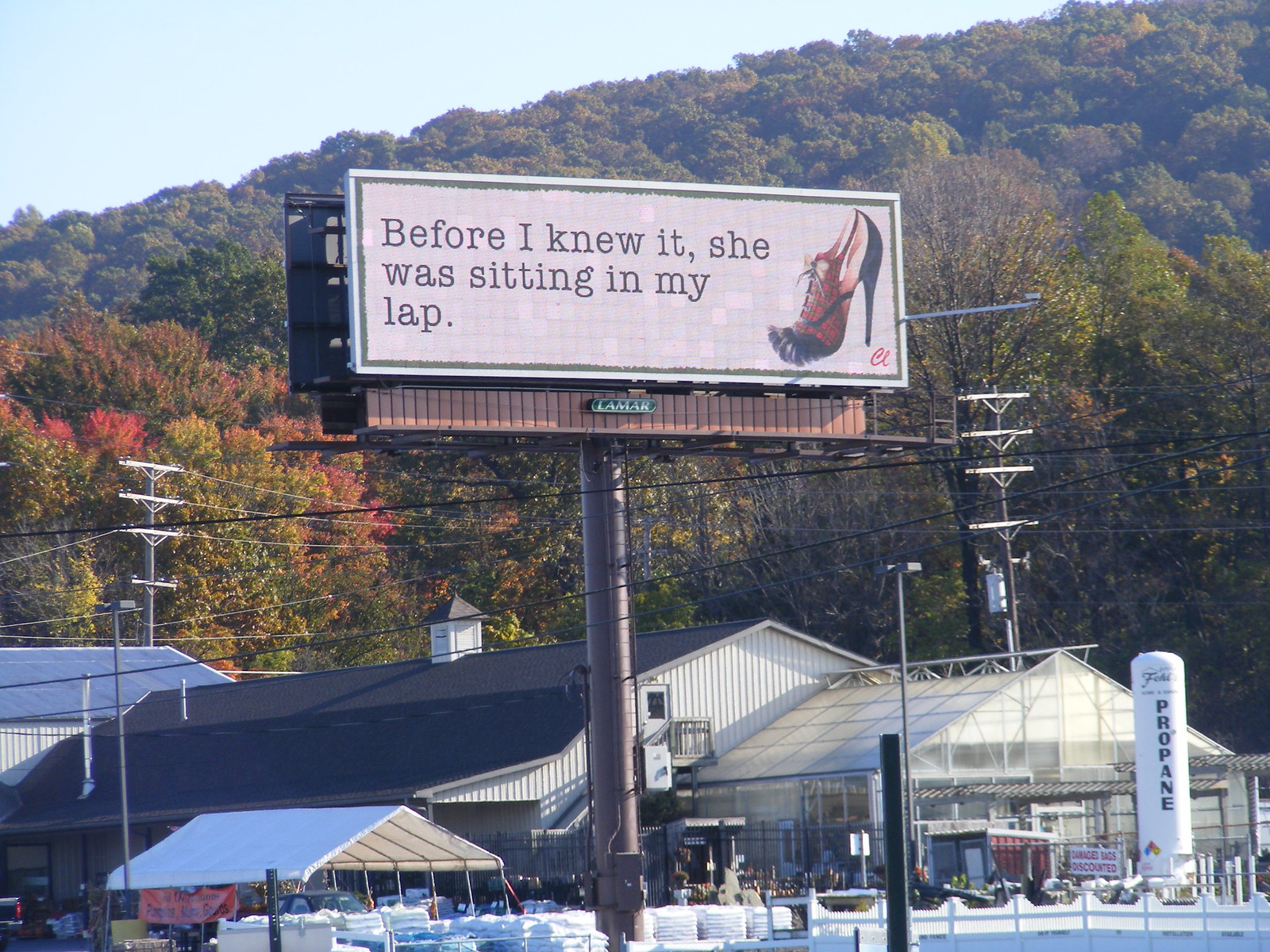This highly detailed square photo features a billboard as the central focal point, slightly angled, displaying the text "Before I knew it, she was sitting in my lap," alongside an image of a high-heeled stiletto shoe and the letters "CL" in red at the bottom left. The billboard, set against a white background with a green border, is mounted on a giant round brown pole. At the base of the billboard is a wooden panel with a green sign that reads "Lamar." Behind this primary billboard, parts of another billboard's backside are visible.

In the distant background, a tree-covered mountain and several power poles with lines extend in various directions. Adding to the pastoral scene, there's a large, rustic building resembling a barn or farmhouse, complete with a small steeple, metal paneling, and a slanted black rooftop. To the right of this structure is a greenhouse and a large white cylinder tank labeled "PROPANE" vertically.

At the lower edge of the frame, stacks of bagged dirt and other white packaged items are visible, indicating an outdoor retail or storage space. The scene is bathed in autumn colors, with reds mixed in among the predominant greens of the foliage, enhancing the blue sky backdrop.